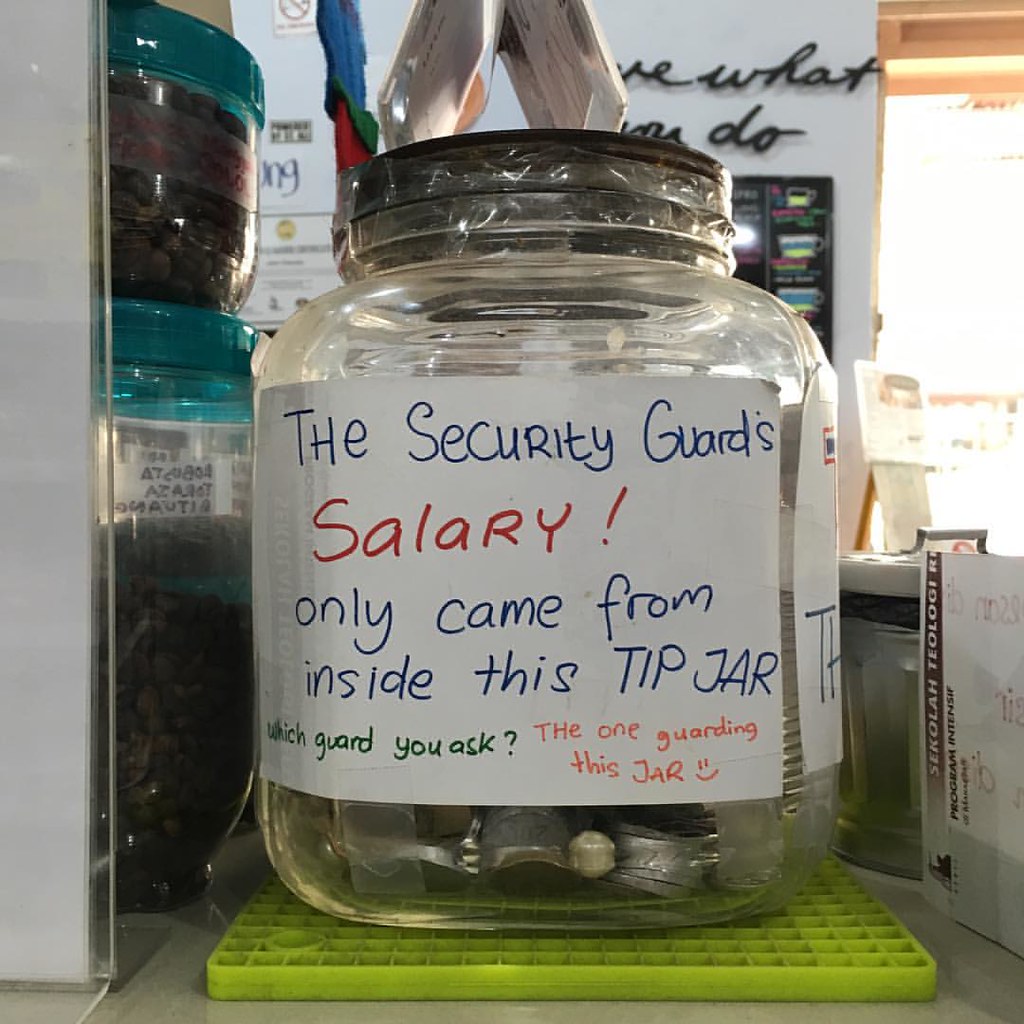This photograph captures a prominently displayed glass tip jar, which is securely taped closed around the rim of its lid, perched on a light green, rectangular mat. The jar is adorned with a white handwritten label bearing colorful, playful text: "The security guard's salary! Only came from inside this tip jar. Which guard you ask? The one guarding this jar 😊." Inside the jar, an assortment of coins and possibly some small trinkets are visible. The setting appears to be inside a store, with the jar positioned on what seems to be a store counter, possibly next to a cash register. In the background, slightly out of focus, are a wall with indistinct details that could resemble a menu, and additional jars with teal-colored lids on the left, presumably containing some form of stored items. The jar is clearly intended to encourage tips for the store's security guard in a humorous and engaging manner.